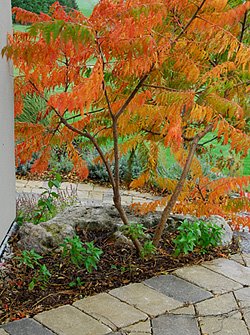This is a detailed photograph of a small, landscaped outdoor area, possibly near the front of a building or home. The focal point is a beautiful tree with two slender stems, boasting vibrant orange leaves that are bunched together, displaying various shades of orange and red. The tree stands in a mulched area that also contains small green plants. The ground features a pathway made of light and dark gray pavers, extending from the bottom right corner to the left. The scene looks slightly damp, suggesting it may have recently rained. The image, presented in a portrait layout, captures the intricate textures and colors of both the foliage and the carefully arranged bricks.